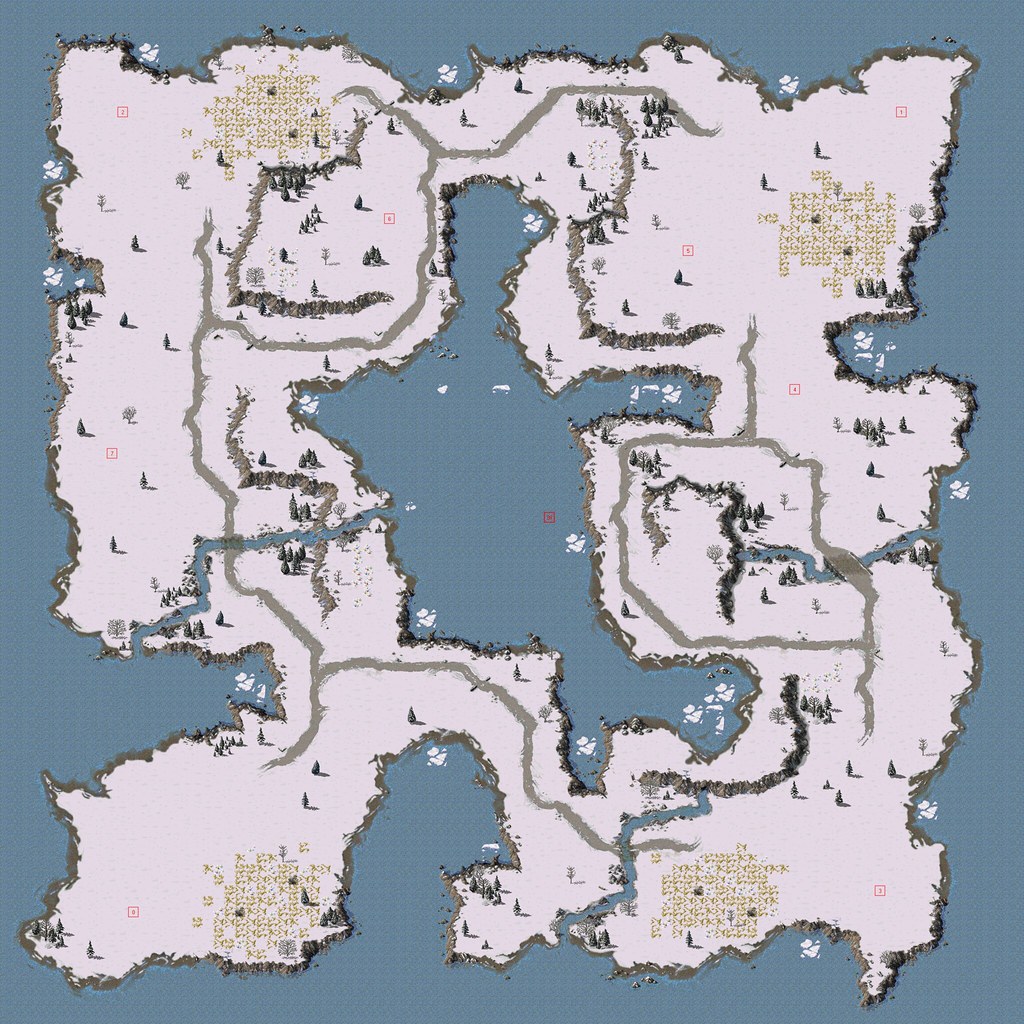This image presents a top-down view of a fantasy map resembling a square-shaped island with irregular, jagged edges forming various inlets, coves, and bays, suggestive of cliffs. The entire island, surrounded by a dark blue expanse of water, is marked by a large central lake dominating the scene. There are multiple gray roads intricately winding throughout the map; one prominent road originates in the top right, meandering around the lake, down to the bottom left corner, and curling further along the southern edge. Another loop of the road can be seen on the right side of the island. The landmass is scattered with numerous trees, illustrated as individual pine trees and green splotches resembling forests or greenery, interspersed with small yellow squares and other topographical features, possibly denoting civilizations, though no discernible structures or towns are visible. The edges of the island have brown, jagged designs evocative of cliffs, enhancing the fantastical nature of the landscape.